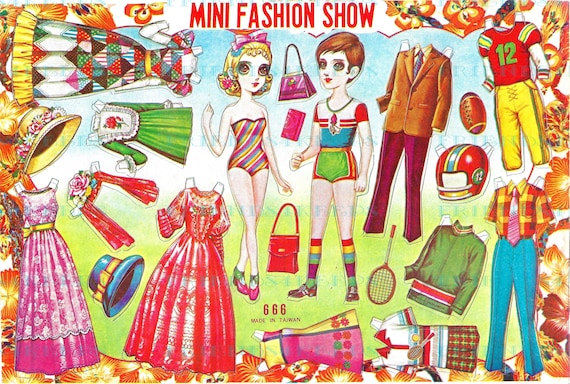This colorful poster, titled "Mini Fashion Show" in bold red lettering at the top, features whimsical paper dolls of a boy and a girl at its center. The girl, sporting short blonde hair adorned with a pink bow, wears a vibrant, rainbow-colored one-piece swimsuit. The boy, with short brown hair, dons a white undershirt with red and blue accents, green shorts with red stripes, and long multi-colored striped socks. Positioned between them are two purses - a red one and a purple clutch. Surrounding the pair are various fashion accessories and outfits: to the left of the girl are an array of dresses and hats, whereas to the right of the boy are items including a suit, a football uniform, a short-sleeved shirt, blue pants, a green jacket, a tennis racket, and a football. Noteworthy details include the inscription "Made in Taiwan" and the enigmatic number "666" at the bottom of the image.